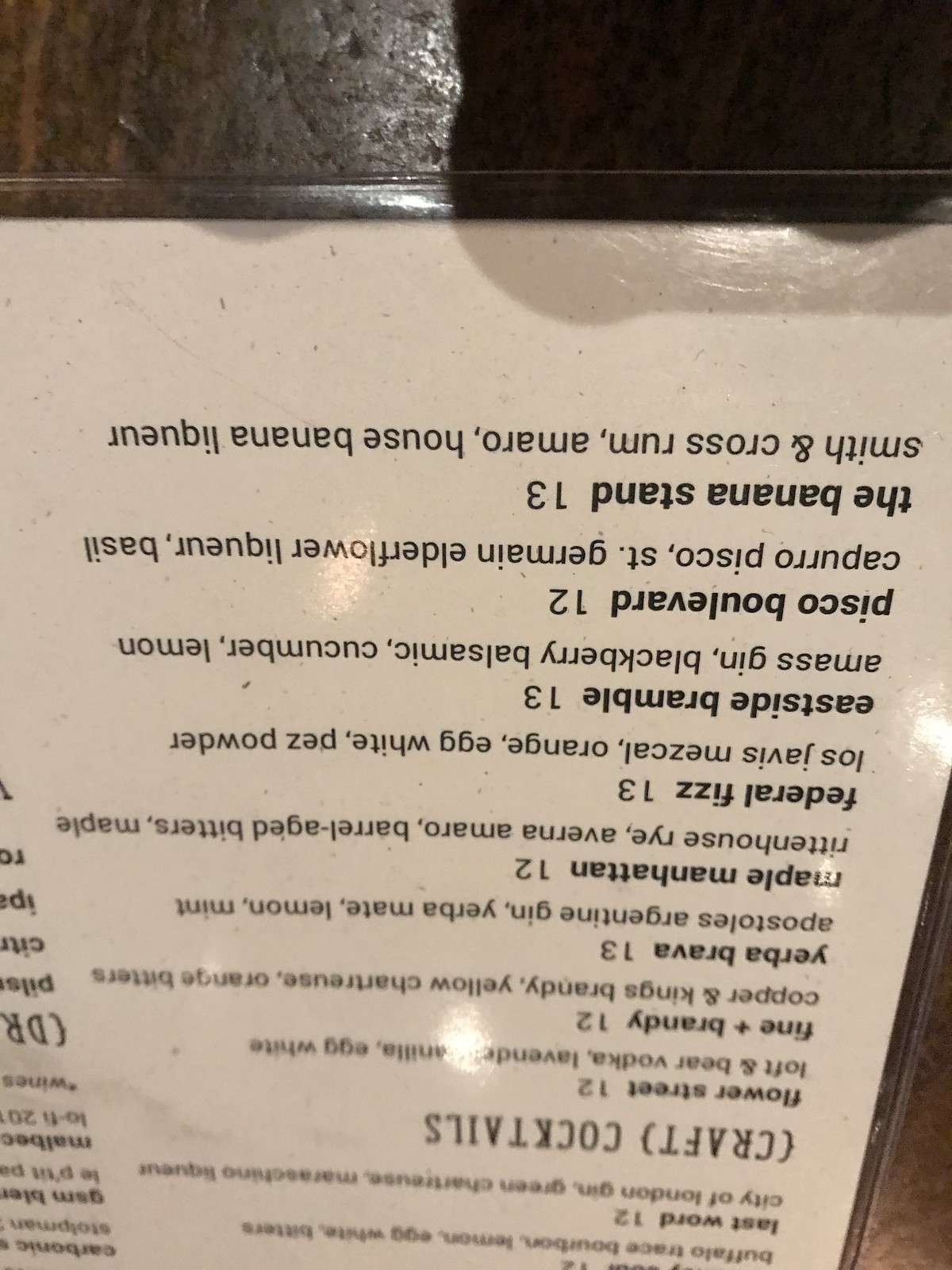This image showcases a cocktail menu positioned upside down on a rustic wooden table. The white, laminated menu stands out against the wooden background due to its transparent plastic covering, which adds a slight sheen. Despite being upside down, the details of the menu are still discernible. The text is printed in black, with each drink name bolded and followed by its price. Descriptions of the drinks are provided below each title in a lighter font. Some of the highlighted items include 'Fine Brandy,' 'Yerda Brava,' 'Feta Fizz,' and 'The Banana Stem.' The entire menu is written in English, offering a detailed insight into the cocktail choices available.